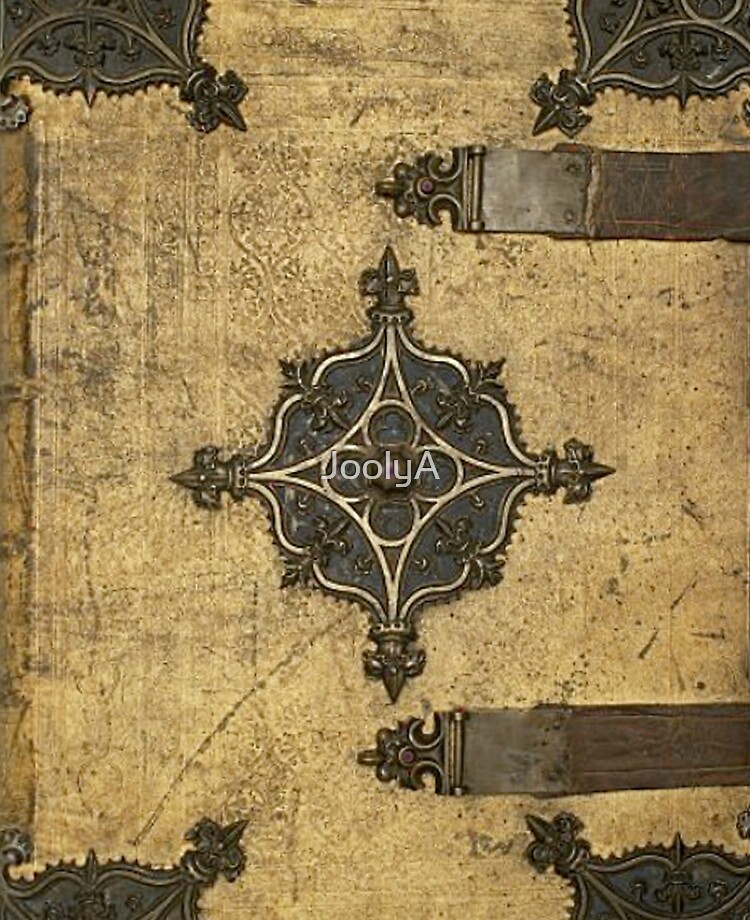The image displays the cover of an exceedingly old book, notable for its ornate design and extensive wear. The cover itself is light brown with darker, scratched areas, giving it a weathered appearance. There are spots and marks all over, suggesting significant age and use. Dominating the cover are metal embellishments: brass emblems at each corner extend several inches inward, each designed in the shape of a crest and featuring rivet details.

The focal point of the cover is a central crest with spikes radiating outward in four cardinal directions, interspersed with smaller spikes. This crest appears black with faded gold outlines. Inscribed in the middle of the crest is the word "JOLLYA" in capital letters. Adding to the book's unique character are two leather straps on the right-hand side, attached with brass points, likely used to secure the book closed. The overall impression is of a book that was once very grand and significant, with intricate details that emphasize its historical and possibly ceremonial importance.